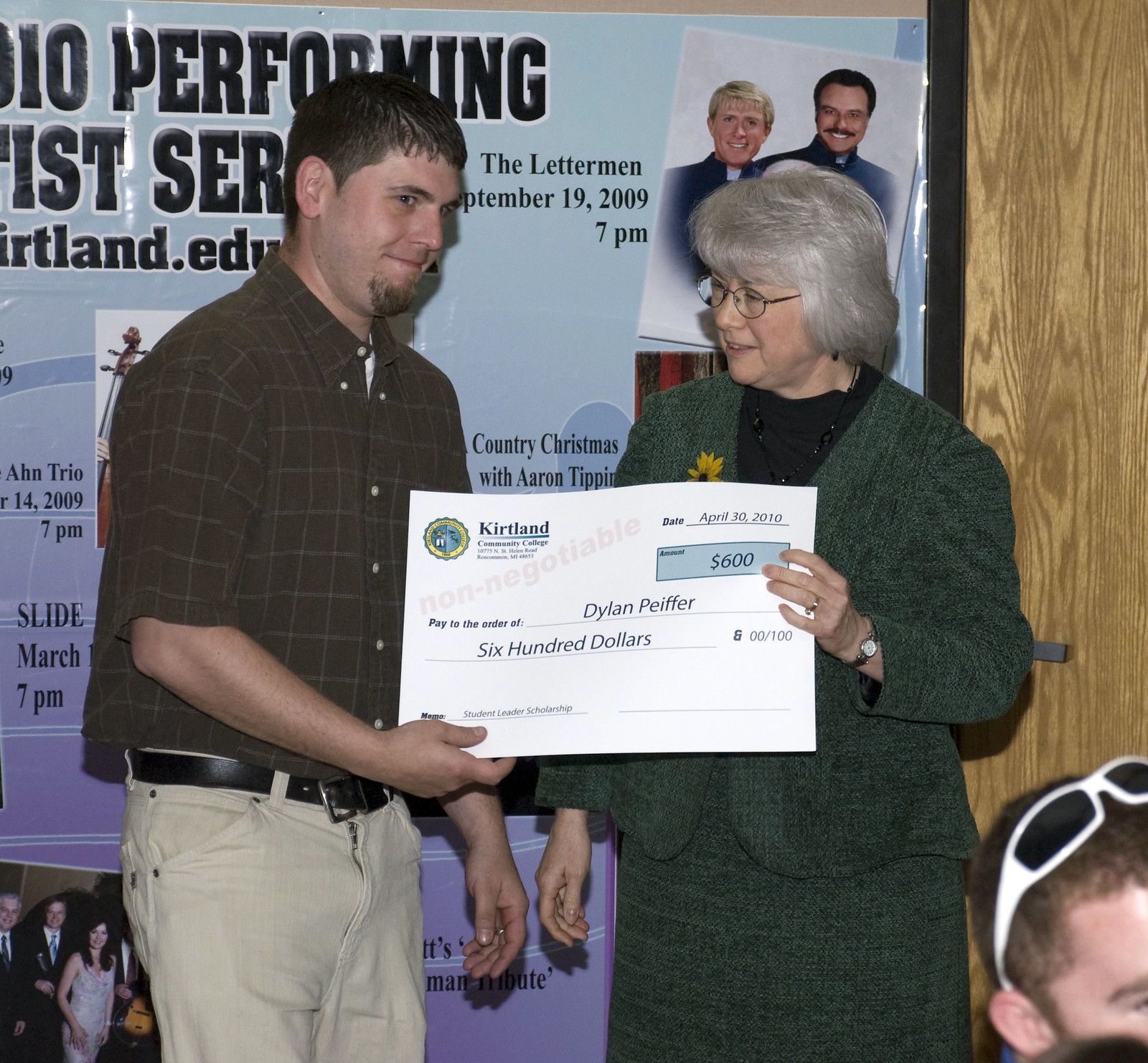In this detailed image, a man with dark brown hair and a short beard stands on the left, wearing a brown and white checkered short-sleeve shirt and khaki pants, accessorized with a black leather belt. He smiles as he holds an oversized check from Kirtland Community College, dated April 30th, 2010, made out to Dylan Pfeiffer for $600. Beside him, an older woman with gray hair, glasses, and a green dress paired with a matching blazer, with a black undershirt, holds the other side of the check. In the background, a partially visible banner on a wooden wall announces an event: it prominently displays "Performing," followed by "The Letterman," with the date September 19, 2009, and the time of 7 p.m. Next to the text is a color photograph of two men, one with blonde hair and the other with black slicked-back hair and a mustache. A few more people can be seen in the bottom right corner of the image. The banner features a light blue and purple backdrop, adding a festive touch to the event, which appears to be a presentation or significant event involving the check handover.